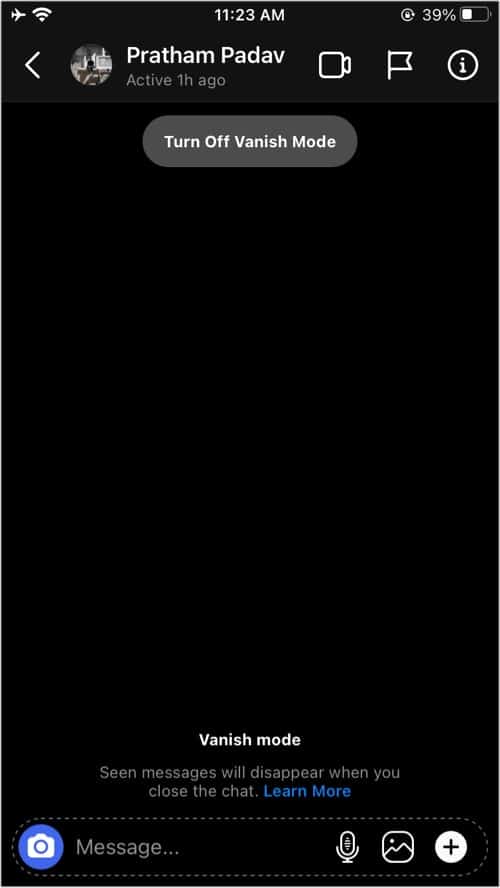This screenshot captures a cell phone interface within an unknown app, possibly a messaging platform. At the top, the user's name "Pratham Padav" is displayed alongside a small profile picture icon. Just below the name, the status reads "active one hour ago." To the right, there are icons for video recording or video chat, followed by a flag and an information icon.

The app appears to be in "Vanish Mode," as suggested by the text "Turn off Vanish Mode" accompanied by a toggle button. The screen is predominantly black, indicating the active Vanish Mode. Additional text clarifies that "Seen messages will disappear when you close the chat," with an option to "Learn more" provided in blue text. 

At the bottom of the screen, a functional bar includes several icons: a picture icon, a central message input area, a voice-to-text icon, an image upload icon, and a plus symbol indicating additional options.